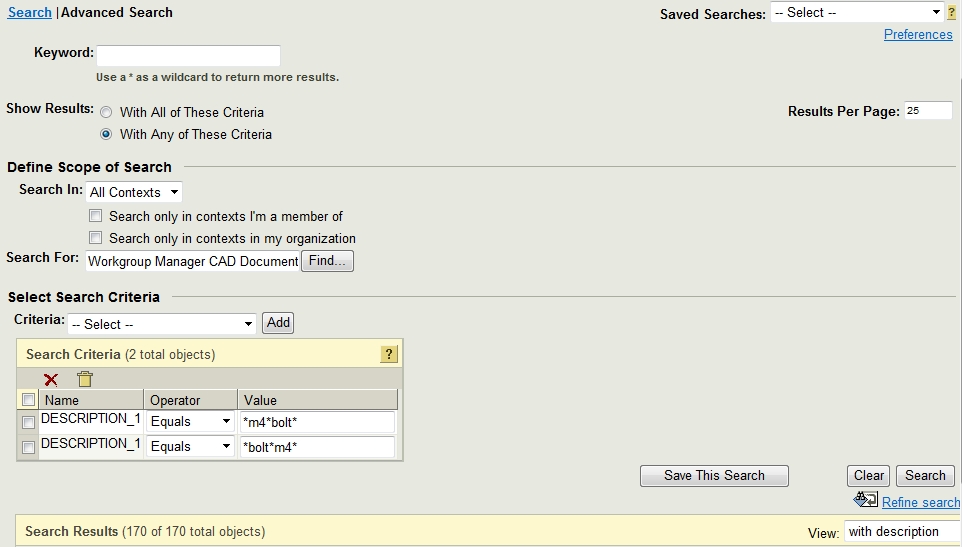**Image Caption:**

The image depicts a search interface page with a slightly gray or manila background. 

- At the top left, the word "Search" is prominently displayed in blue, adjacent to "Advanced Search" written in black.
- On the top right, a drop-down box labeled "Save Searches" is visible, offering a "Select" option and a help icon (question mark) to its right. Next to these, a blue "Preferences" button is present.
  
The central area of the interface is structured as follows:

1. **Keyword Search Section:**
   - "Keyword" is written in black, just above a white input box.
   - Below, it states: "Use an asterisk (*) as a wildcard to return more results."
  
2. **Criteria Selection:**
   - Two buttons are listed to determine search criteria:
     - The top button (unselected) says "Show results with all these criteria."
     - The bottom button (selected) says "Show results with any of these criteria."
  
3. **Results Per Page:**
   - Set to "25."

4. **Scope of Search:**
   - Options include:
     - "Search in all contexts."
     - "Search only in contexts I’m a member of."
     - "Search only in the context of my organization."
   - All checkboxes are currently empty.
  
5. **Additional Search Filters:**
   - Options for searching specific categories such as "Work Group Manager CAD Document" are present.
   - There is a "Find" button associated with these filters.

6. **Search Criteria Selection:**
   - Text options labeled "Search Criteria," and a drop-down box titled "Criteria" with an "Add" button are available.
   - A section showing "Search Criteria: 2 total objects" details parameters such as:
     - Description 1: "M4 Bolt"
     - Description 2: "Bolt M4"
  
7. **Search Results:**
   - Indicates "Search results 170 of 170 total objects."
   - Below this, there are three actionable buttons: "Save the Search," "Clear," and "Search."

The layout is detailed, offering multiple ways to refine and define search parameters effectively.